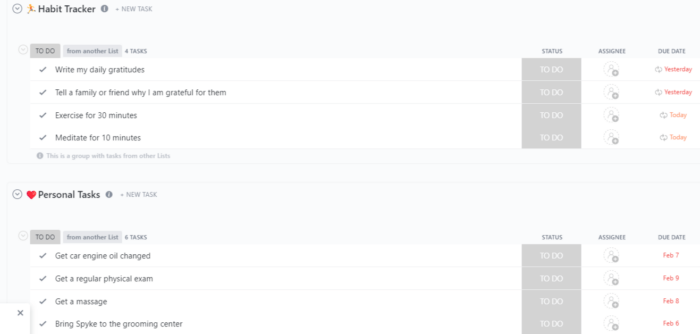The image depicts a digital personal organizer with two distinct columns and a blank space in the center. 

On the left-hand side, there's a segmented layout. The top segment is labeled "Habit Tracker" and features an illustration of a person running. Beneath this, it lists various actionable items such as "To Do: Check this, check that, check the next thing." The second segment is titled "Personal Tasks," containing specific errands like "Get car engine oil changed" and other miscellaneous tasks.

The right-hand column lacks explicit titles but contains sections for "Status," "Assignee," and "Due Date." For example, one entry indicates a Status with a time stamp at 10:00 am, an Assignee labeled "10:00 am," and a Due Date of the previous day. Another section in the same column lists dates in a non-sequential order: February 6th, 7th, 8th, and 9th, suggesting a jumbled arrangement rather than chronological order.

Overall, the organizer merges elements of a habit tracker and task manager, providing a comprehensive overview of personal tasks and their statuses.